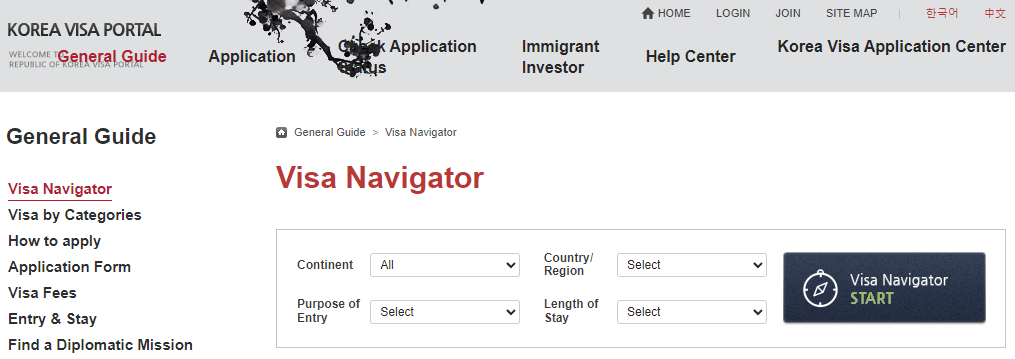The image features a comprehensive layout for the Korea Visa Portal. At the top, there is a light gray rectangle with "Korea Visa Portal" written on the left. Below this are various words in black, overlaid with red text. The red text reads "General Guide" followed by "Application." Adjacent to this is an image resembling a branch with leaves. The word "Application" appears again next to the branch icon. 

In the top right corner, there is an image of a house labeled "Home," accompanied by "Login," "Join," and "Site Map." Below these elements, a small gray line runs across the screen, followed by Asian characters in red. Underneath these characters, it says "Help Center" and "Korea Visa Application Center."

On the left side of the image is another section labeled "General Guide" in black, with "Visa Navigator" underlined in red beneath it. The list of topics under this section includes "Visa by Categories," "How to Apply," "Application Form," "Visa Fees," "Entry and Stay," and "Find a Diplomatic Mission."

To the right, there is a gray square containing some indiscernible white text. Below it, a section marked "Visa Navigator" is followed by a series of rectangles outlined in gray. Each rectangle has words and an arrow pointing downward next to it. The first rectangle says "All," while the subsequent rectangles simply say "Select" with a downward arrow. 

Further down is a blue rectangle with a symbol consisting of a circle and an oval shape. This rectangle also reads "Visa Navigator" in white, followed by a green button labeled "Start."